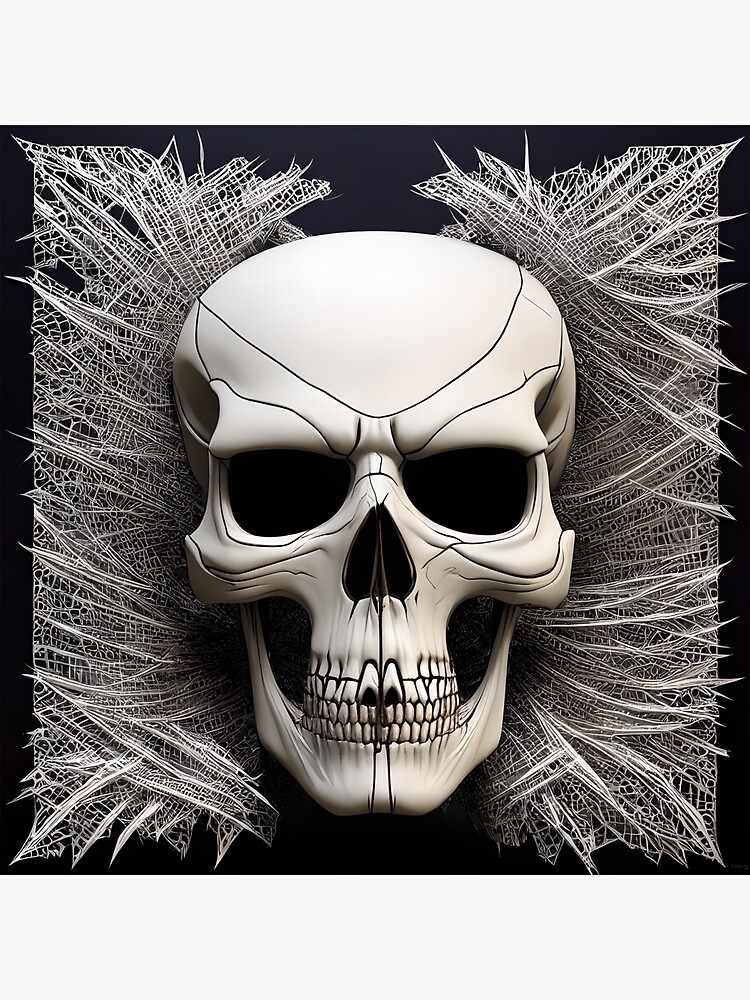The image portrays a detailed, close-up 3D render of a human skull, appearing almost plastic or silicone-like in its smooth, reflective texture. Dominating the center, the skull is a stark white contrasted against a predominantly black background. A striking feature is the intricate network of fine black lines that meticulously trace the skull, especially accentuating the divide from the nose down to the chin, and forming rounded patterns over the forehead and temporal lobes. This creates a sense of depth and segmentation across the skull's surface.

The skull's eye sockets and nasal cavity are deep black, creating an eerie void, and the teeth are prominently visible with an extra row on the upper jaw, adding an unsettling layer to its anatomy. Below the main row of teeth, a defined split under the nose diverges into two distinct lines stretching toward the corners of the chin.

Surrounding the skull, a series of dense, white fibers or spiderweb-like formations create a symmetrical pattern that expands outward to both the left and right sides, some even extending beyond the black border that frames the image. Above the skull, this web-like texture is subtly tinged with purple, providing a stark, otherworldly contrast against the primary black backdrop. This intricate render creates a hauntingly mesmerizing visual, blending detailed anatomical depiction with abstract, web-like complexities.